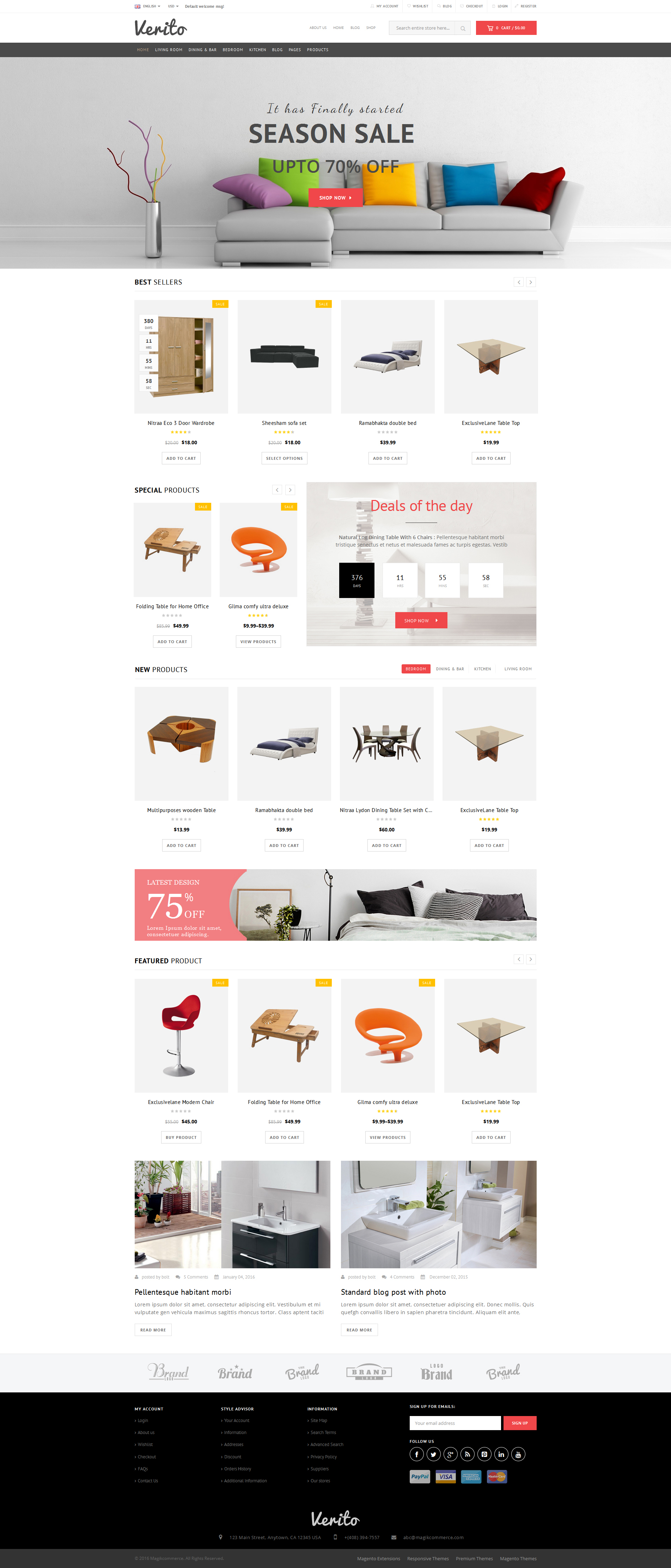**Detailed Description of the Home Furnishing E-commerce Website**

The website presented is an online store dedicated to home furnishings, believed to be named "Burrito" based on its stylized VRITO logo. The site is designed with usability in mind, offering features and information in a structured layout:

- **Header Information**: 
   - The top section includes a drop-down menu for changing the currency and language, defaulting to USD and English.
   - To the right, there are tabs for "My Account" and another unreadable tab, followed by the "Checkout" button.
   - Beneath these, a search bar is positioned next to the red "Cart" icon.

- **Main Navigation Menu**:
   - Located beneath the logo, the primary navigation bar spans the width of the website. It includes categories such as Home, Living Room, Dining, Bar, Bedroom, Kitchen, Blog, Pages, and Products.

- **Central Banner**:
   - A prominent graphic showcasing a gray L-shaped sectional with multicolored pillows dominates the center of the homepage. This section promotes a seasonal sale with discounts up to 70% off, accompanied by a "Shop Now" call-to-action button.

- **Featured Products Section**:
   - Below the banner, a carousel of bestsellers is displayed, featuring a variety of home furnishings. Notable items include:
     - **Nitro Echo Three-Door Wardrobe**: Rated 4 out of 5, priced at $318 (original price struck through), with an “Add to Cart” option.
     - **Sofa Set**: Available for $418, with a “Select Options” button.
     - **Double Bed**: Priced at $399.99.
     - **Tabletop**: Selling for $20, labeled as a special product.
     - **Deal of the Day**: Features a natural log table with six chairs.

- **Product Filters and New Products**:
   - Users can filter products by room categories, including Bedroom and Dining. 
   - New products are prominently listed, encouraging exploration of the latest designs.

- **Footer Section**:
   - This section highlights additional features such as:
     - Latest designs at 75% off.
     - Featured products displayed in four distinct images.
     - Blog links for further reading.
     - An email signup form for newsletters.
     - Information on accepted payment methods and social media follow options.

This comprehensive, user-friendly design ensures that customers can easily navigate and find the perfect items for their home furnishing needs while taking advantage of promotions and new product offerings.